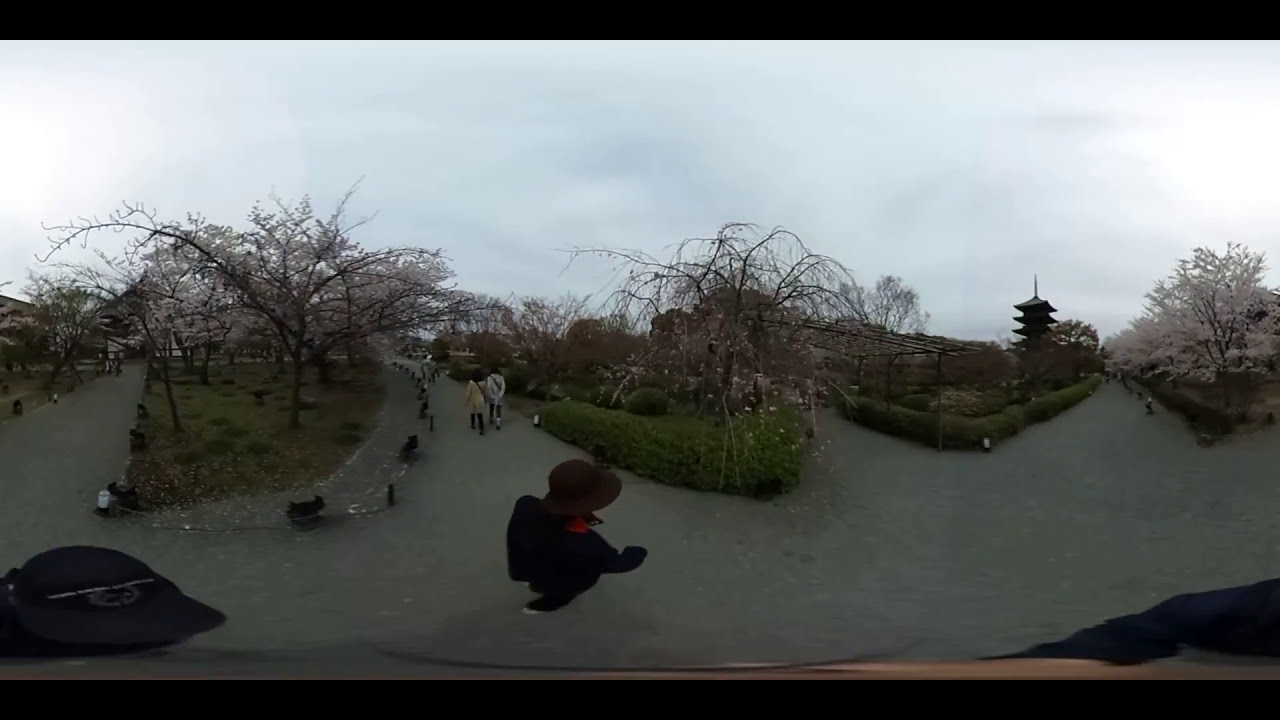In this color photograph, taken through a fisheye or barrel-distorted lens under a grayish, overcast sky, we see an early spring garden scene. The image has a horizontal black stripe across the top and bottom and is in landscape orientation. A person, viewed slightly from above, stands in the foreground wearing a broad-brimmed burgundy hat and a long-sleeved black jacket. The garden is divided into multiple grassy islands, each bordered by gray pebble paths. There are numerous trees with budding pink flowers, resembling cherry blossoms, yet to fully leaf out. People stroll along various paths; notably, two figures can be seen wearing cross-strap shoulder bags. In the bottom left, a baseball cap and a black dog are visible. Towards the upper right, an Asian-style pagoda with multi-tiered roofs and a tall central spike stands prominent. The color palette of the photo is murky and subdued, contributing to the scene’s serene yet surreal atmosphere.